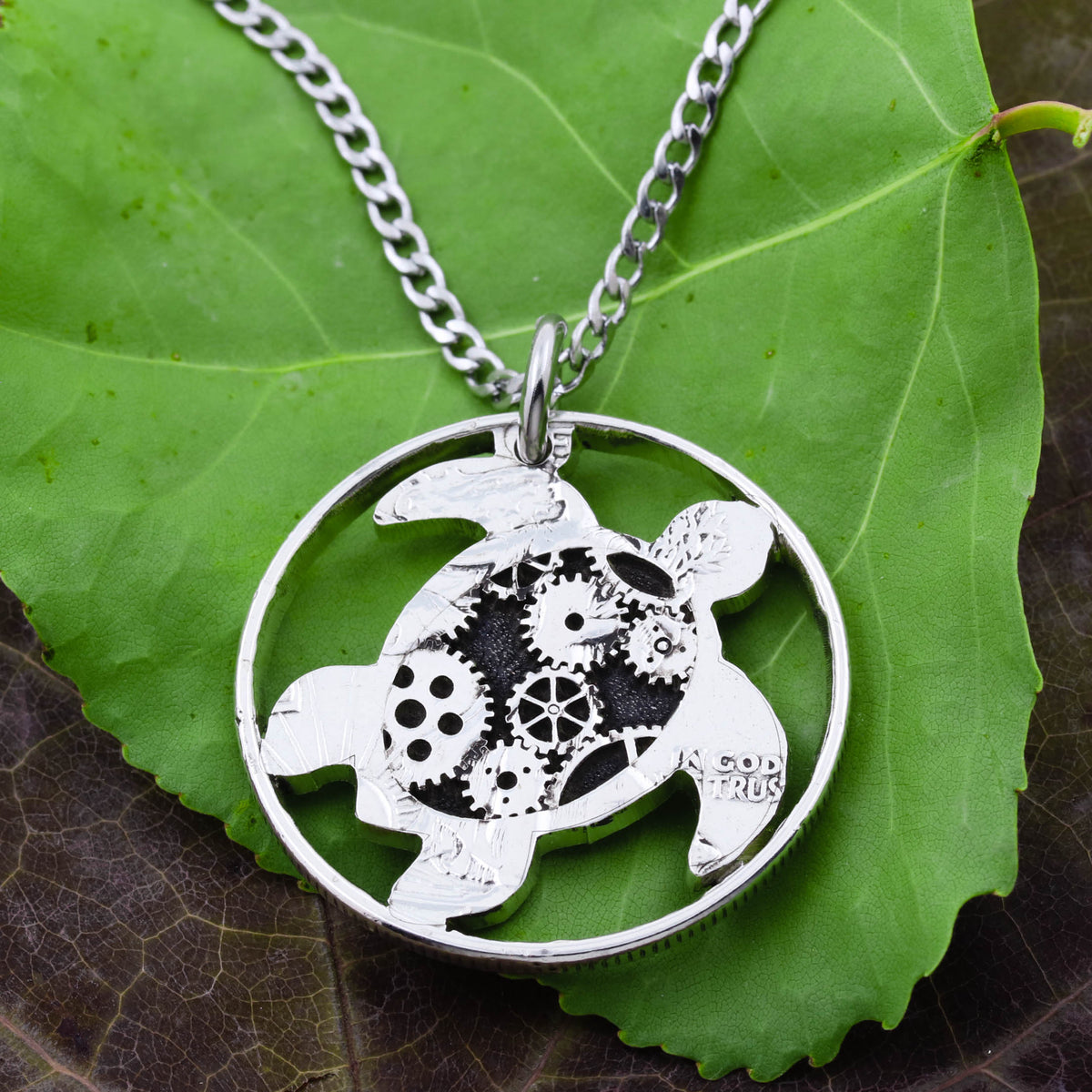This detailed color photograph showcases a unique pendant, expertly crafted from what appears to be a coin, suspended from a robust silver chain that suggests a men's necklace. The pendant is circular, encasing a meticulously designed silver sea turtle. Notably, the right flipper of the turtle bears the partial inscription "God We Trust," indicating its origin from a coin. The turtle's shell is adorned with intricately meshed gears, set against a striking black background, reminiscent of steampunk design elements commonly found in watches. The pendant is artfully displayed on a vibrant green leaf, which rests atop a darker, almost black leaf, emphasizing the contrast and the intricate details of both the turtle and the gears within.